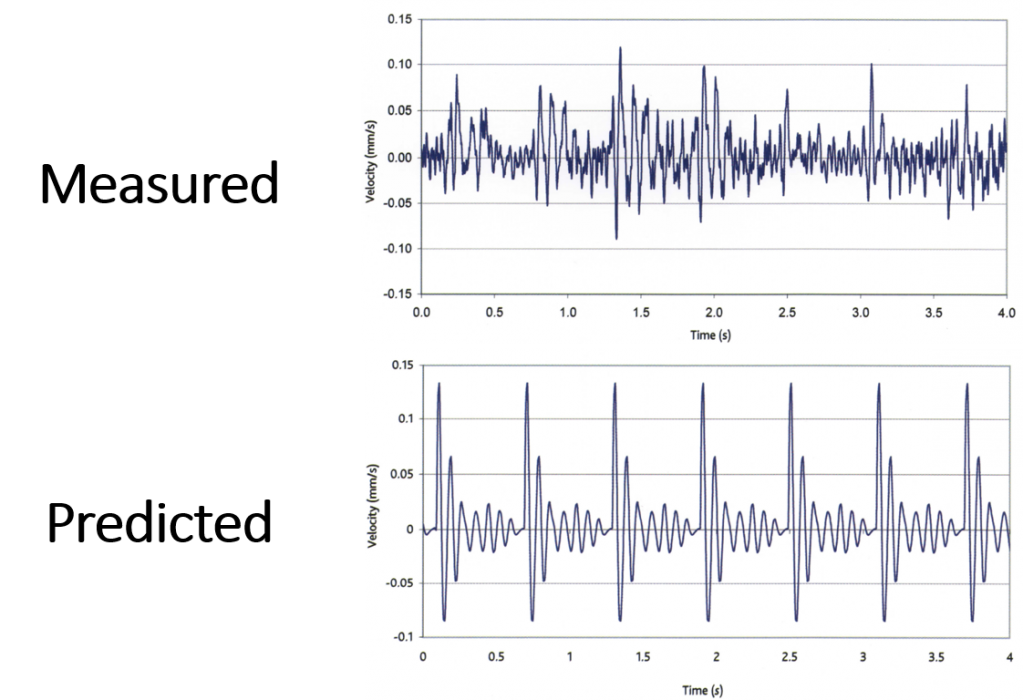The image showcases two adjacent charts stacked vertically, each with a white background. The top chart is labeled "Measured Velocity" and displays a graphical plot reminiscent of a heartbeat monitor, where velocity is mapped against time. The left side of the graph marks the velocity increments in values such as 0.05, 0.10, and 0.15, while the bottom axis measures time, incremented by 0.5 units. The squiggly line representing the measured data fluctuates tightly across the graph. 

Below it, the second chart, labeled "Predicted Velocity," uses the same axes and increments as the top chart. However, the visual data shows a less dense pattern, with more spread-out, elongated squiggles compared to the measured graph. Although the measured and predicted velocities are plotted similarly, notable differences are observed, indicating slight disparities between the actual measurements and the predictions.